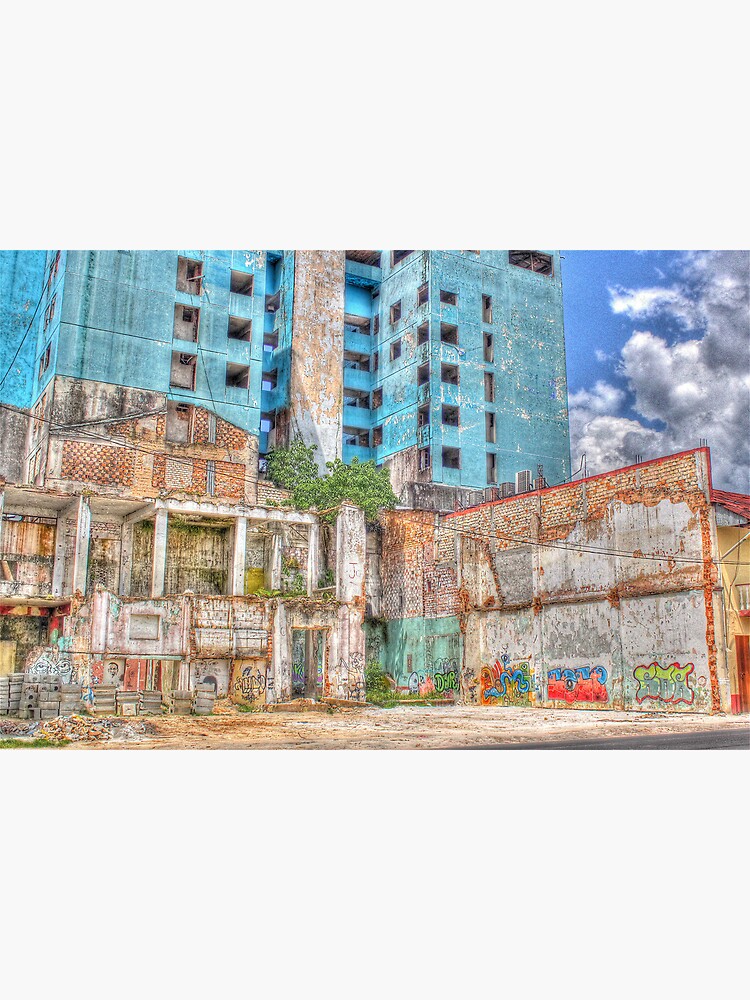The image depicts a stylized, possibly digitally altered representation of a rundown neighborhood, likely a favela or barrio from a poorer country. The central focus is a heavily graffiti-covered building or wall made of bricks and concrete that appears poorly maintained, adorned with bright colors due to heightened saturation and contrast, lending it a somewhat cartoonish and unrealistic look. The building, resembling old, possibly Eastern European architecture, is partially obscured by a growing tree and moss, suggesting abandonment. Additionally, the image captures a detailed mural that incorporates three-dimensional elements of bricks, pillars, and stones, evoking the facade of a decrepit building. The backdrop features a blue sky with white fluffy clouds, while the ground appears to be dirt, enhancing the sense of decay and neglect.